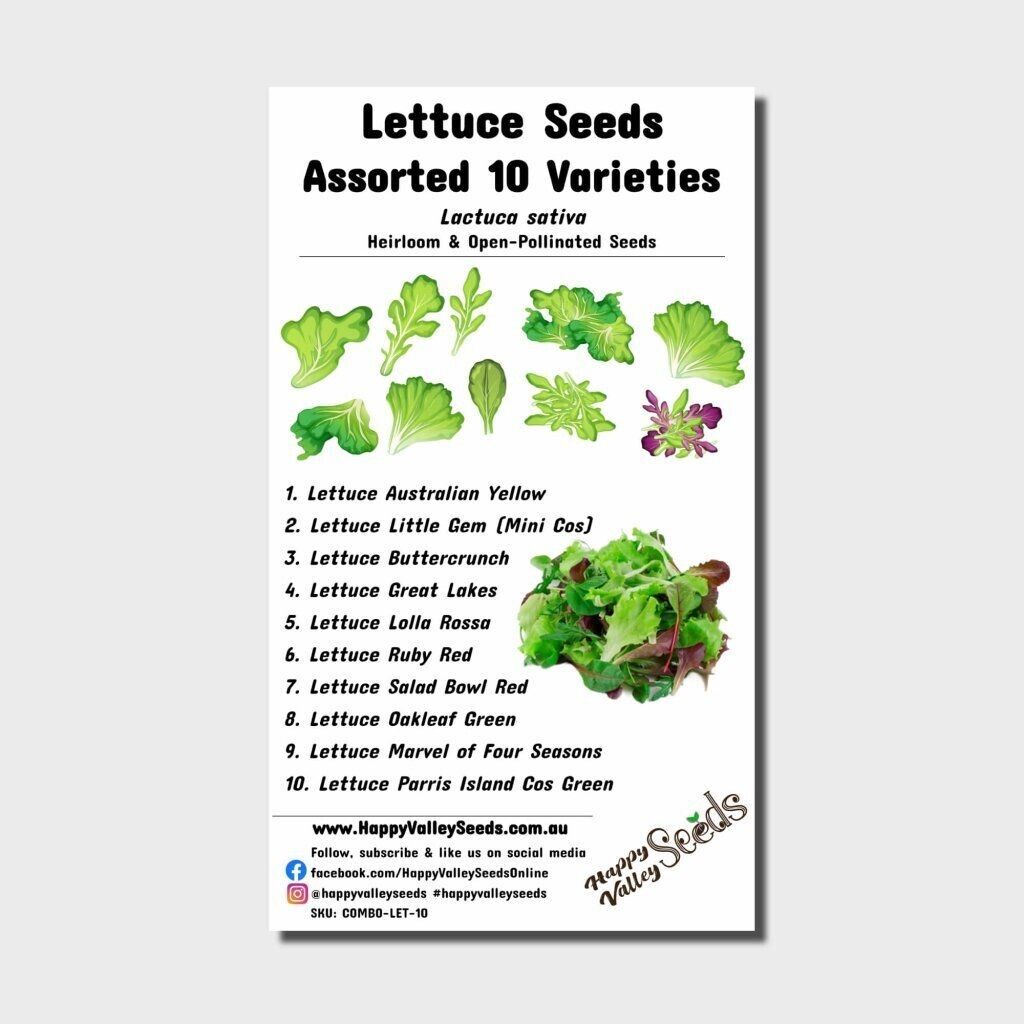This is an infographic poster about lettuce seeds, featuring the title "Lettuce Seeds" at the top in black text, followed by "Assorted 10 Varieties" and "Lactuca sativa." Beneath that, the poster states that the seeds are heirloom and open pollinated. A horizontal line separates the title section from the main content. 

The main content showcases two rows of images, each containing five pictures of different lettuce leaves, representing the ten varieties. Alongside the images, there is a numbered list of the lettuce varieties, including:

1. Australian Yellow
2. Little Gem
3. Buttercrunch
4. Great Lakes
5. Lola Rosso
6. Ruby Red
7. Super Salad Red
8. Oak Leaf Green
9. Marvel of Four Seasons
10. Paris Island Cos Green

To the right of the list, there is an illustration resembling the head of a cabbage, composed of various lettuce leaves.

At the bottom of the poster, another horizontal line separates the main content from the footer, which includes the URL www.happyvalleyseeds.com.au, and social media prompts. The footer features a Facebook icon with a link, an Instagram logo with the corresponding username, an SKU number, and the stylized text "Happy Valley Seeds" rising diagonally from left to right.